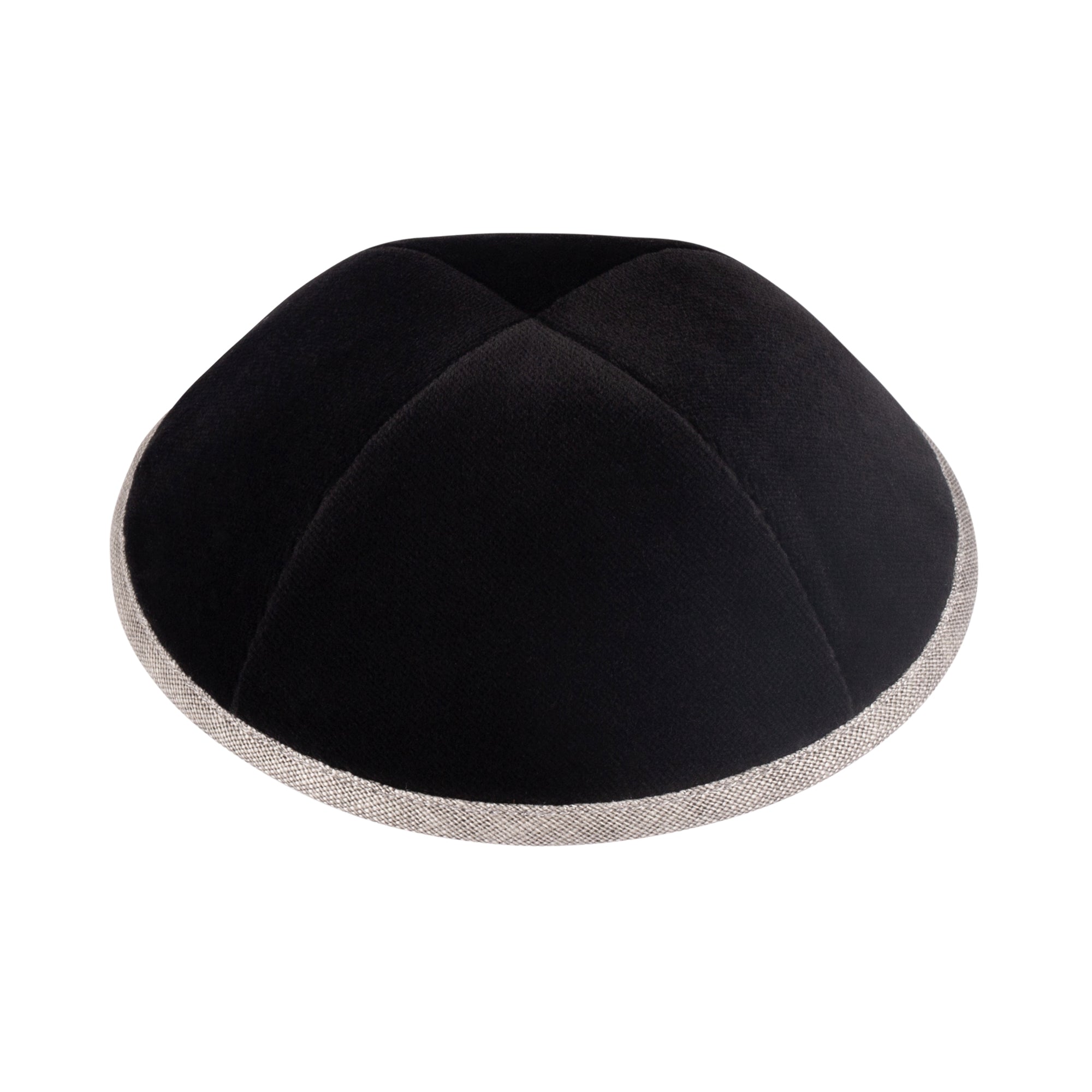In this photorealistic image, we observe a small black cap resembling a yarmulke. The cap is made of black fabric with a distinctive pleat at the very center, giving it a slightly raised, three-dimensional form. It's constructed from four wedge-shaped segments sewn together. A striking feature is the white or light gray linen fabric lining its bottom circumference, adding a defined border. The cap exhibits a central seam running from the bottom to the top, intersecting perpendicularly with another seam, meeting at the very top. The top of the cap appears slightly concave, as if gently pressed down. The background of the image is flat white, providing a stark contrast to the cap, which allows its detailed construction and textures to stand out.